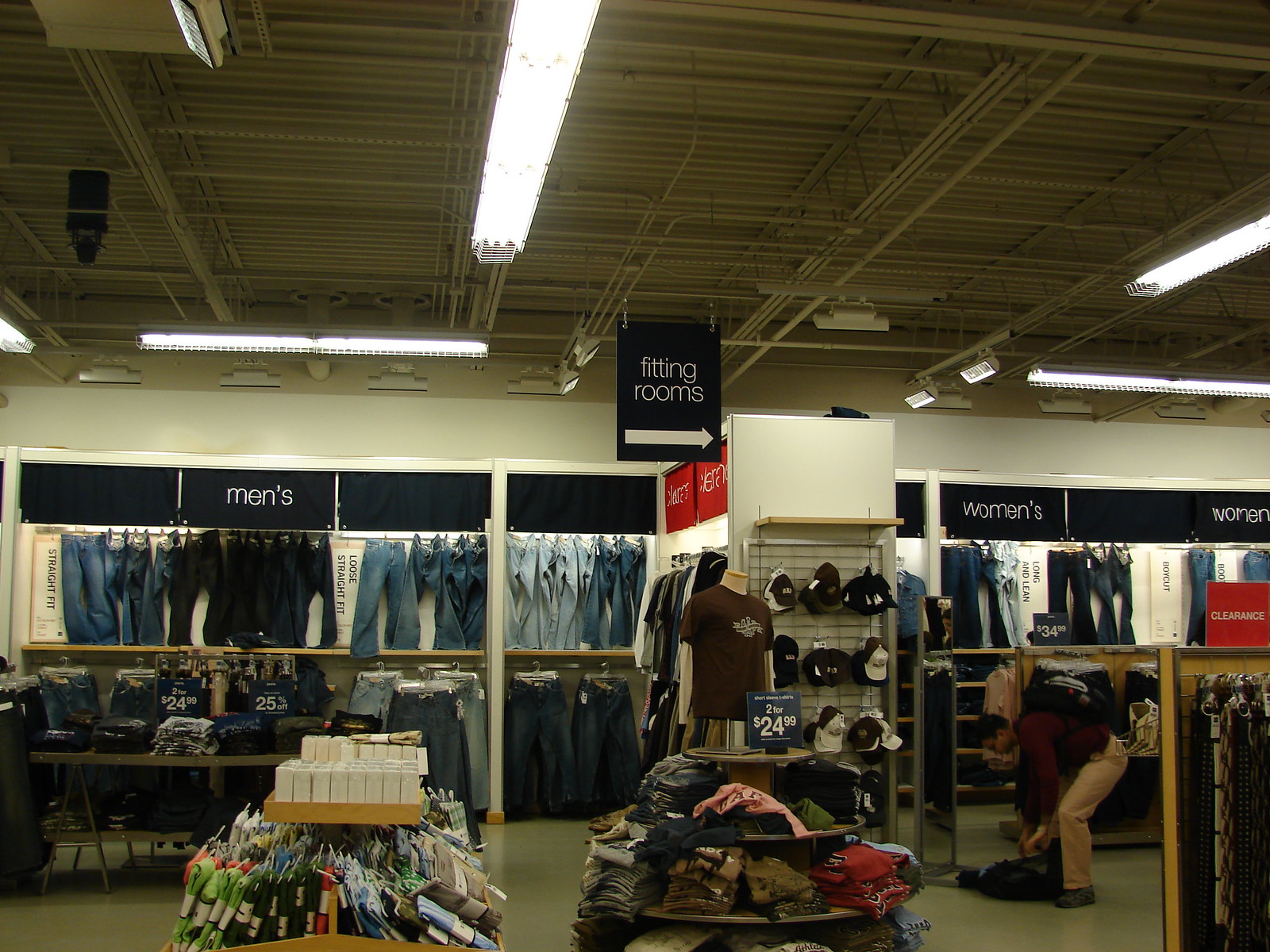Inside a retail clothing store with an industrial tan-painted metal ceiling and illuminated by long fluorescent light tubes, the store is distinctly divided into men's and women's sections by a central pillar. The pillar is adorned with a wire grid showcasing various colored baseball caps, including burgundy, black, and burgundy with white fronts. The men's section on the left, indicated by a black sign with white "MEN'S" lettering, features an assortment of jeans in different shades of blue and black, hung in beige cubbies with metal rods. Similarly, the women's section on the right, marked by a matching "WOMEN'S" sign, displays darker jeans graduating from dark blue to lighter blue shades.

In front of the central pillar, a circular table with four progressively smaller shelves is laden with t-shirts and a sign reading "2 for $24.99." Additional promotional signs, such as "25% off" and "$34.99," can be seen around the store. A red clearance sign marks the clearance section on the women's side. Among the shoppers, a man is seen interacting with his backpack on the floor, possibly trying on some clothes.

The fitting rooms are also located on the right side, indicated by another black sign with an arrow pointing the way. The store's organized layout combines functional and aesthetic elements to cater to various shopper needs, making it a comprehensive retail environment.